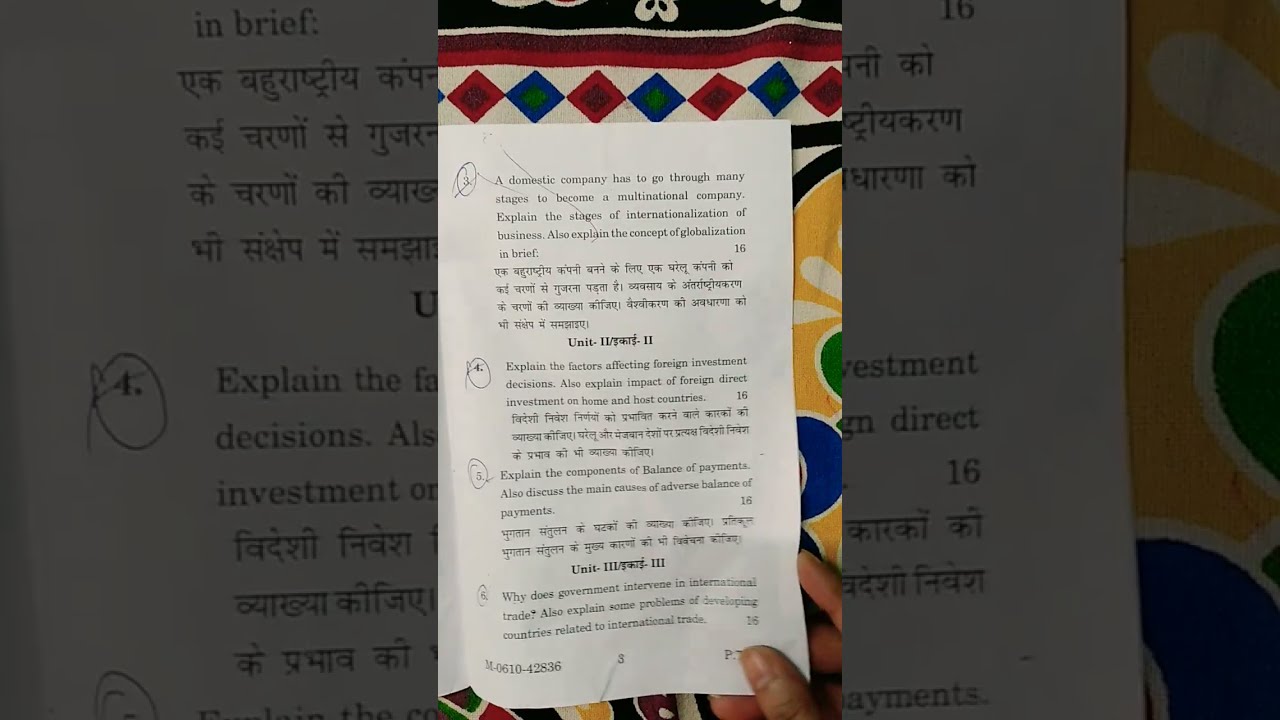This image features the partial view of an educational document, centrally displaying text in both English and a foreign language. The visible content includes questions about economic topics such as the stages of internationalism, globalization, and factors affecting foreign investment decisions. The paper is held at the lower right corner by three fingers, with the holder having darker skin. Surrounding the text is a vibrant, colorful blanket adorned with alternating red and blue diamonds along the top, interspersed with green diamonds in the center, and red, white, and maroon stripes. The right side of the blanket features a yellow circular pattern with a black edge and white flowers, alongside other green and blue elements. Notably, part of the document is cut off by another overlaid piece of paper. The bottom left of the test paper reveals a circled number four and sections of text, indicating missed answers. The image composition gives the impression that the paper is resting on a visually striking cloth, likely a tablecloth or blanket, enhancing the academic work with a burst of color.